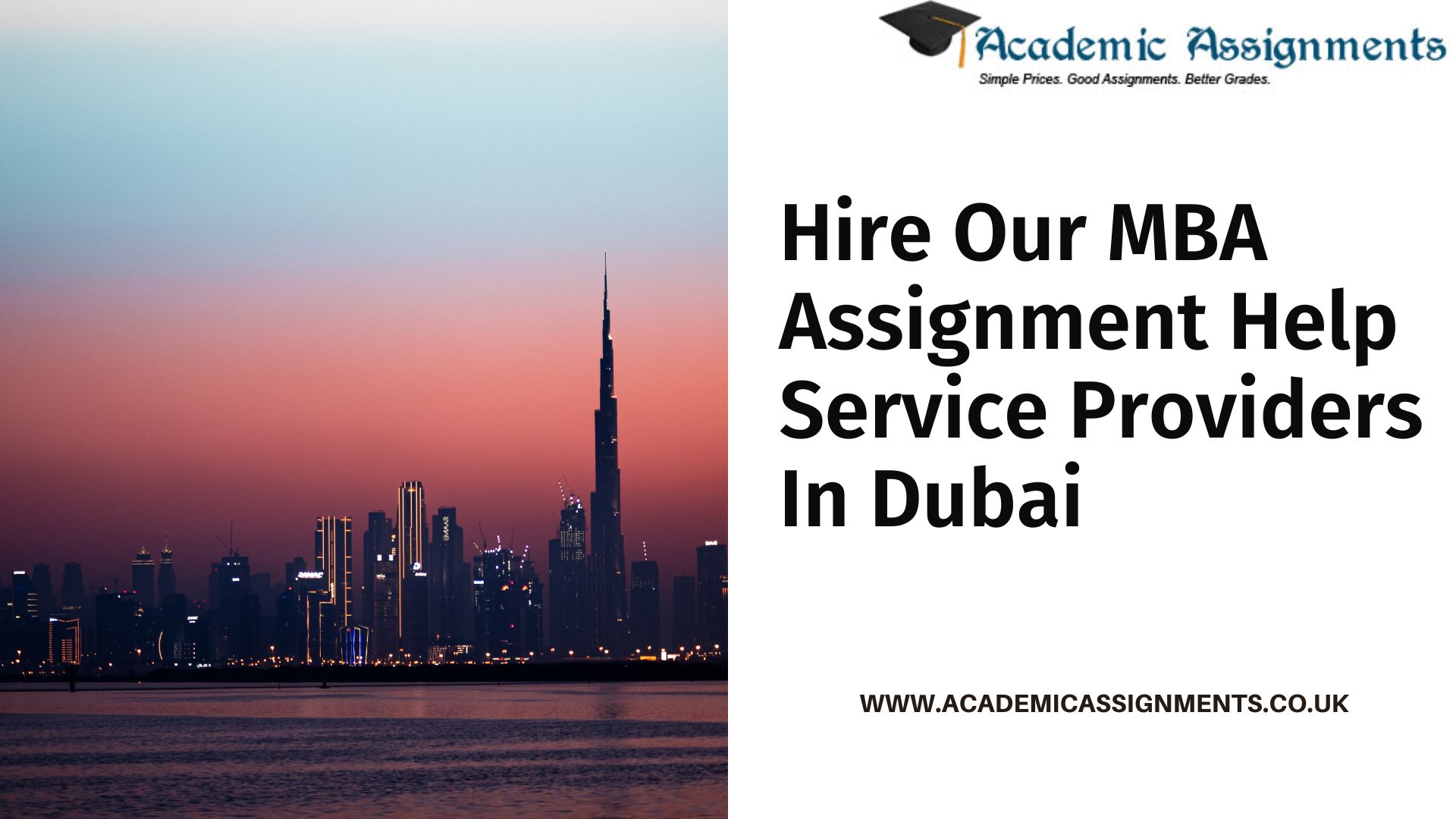The image is a screenshot from a computer, featuring a split layout with a photograph on the left and text on the right, set against a white background. The photograph depicts a city skyline at night. The sky at the top of the image transitions from blue to an orange-red hue. A row of buildings stretches from left to right, punctuated by a tall, pointed skyscraper on the far right that reaches into the blue part of the sky. In the foreground, a body of water reflects the cityscape.

On the right side of the image, the upper-right corner features a blue background with the text "Academic Assignments" accompanied by an icon of a black graduation cap to its left. Below this, the tagline reads "Simple prices, good assignments, better grades." Further down, in bold text, it states, "Hire our MBA assignment help service providers in Dubai." There is a small white gap followed by the website URL "www.academicassignments.co.uk." The bottom of the right section is left blank, creating a balance with the dense information above.